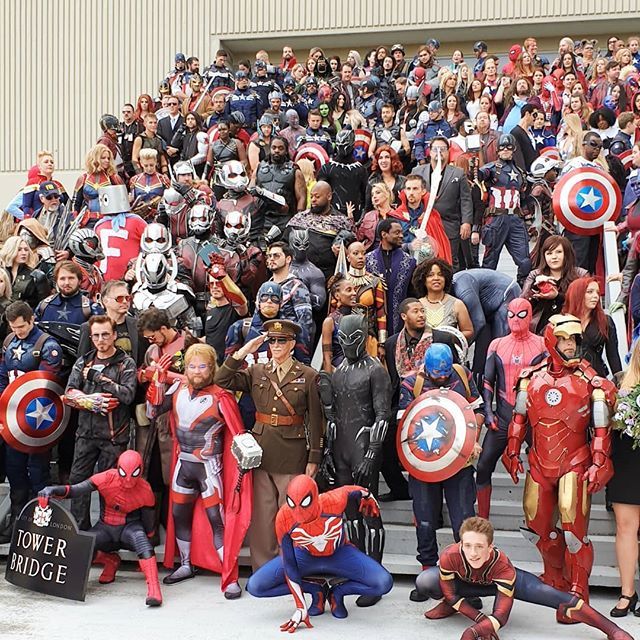A large group photo features a diverse assembly of individuals dressed as various Marvel characters. The image showcases a myriad of Spider-Men, each donning different costumes from various Spider-Man iterations, alongside multiple renditions of Iron Man, Captain America, Ant-Man, and Thor. 

In the front row, starting from the left, we see Captain America, followed by a character resembling the Hulk, then Spider-Man kneeling down, a version of Thor, Black Panther, another Captain America, and Iron Man. Three Spider-Men are positioned prominently in a kneeling pose in the front.

Behind this front row stands a plethora of Marvel characters arranged on bleachers. Among them are Doctor Strange, Black Widow, Scarlet Witch, and Captain Marvel, along with many others, all contributing to the vibrant tableau of Marvel's iconic heroes and villains. The scene is a colorful and dynamic celebration of the Marvel universe, with characters intricately arranged to capture the spirit of their respective personas.